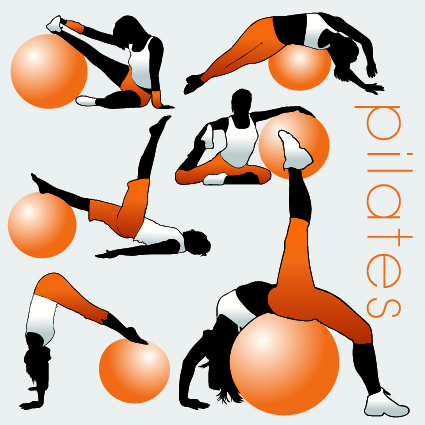The image is an informational graphic about Pilates set against a light gray background. The word "Pilates" is written vertically in lowercase letters in an orange hue along the right side. The graphic showcases six cartoon-like drawings of a silhouetted woman wearing a white tank top, orange leggings or shorts, orange wristbands, and white sneakers. The woman's body is rendered entirely in black. She is depicted performing various Pilates exercises using a spherical orange exercise ball, highlighted with white where the light hits it.

- In the upper left, she is sitting on the ground with her right leg resting on the ball, holding her foot with her right hand.
- To the right of this, she lies sideways on the ball, her feet on one side and her hands on the other.
- Below that, she sits on the ground with her left leg stretched up behind her and her left arm balanced on the ball.
- In the bottom left, she performs a partial handstand, with her hands on the floor and her feet resting on the ball.
- Beside this, she lies on her back, her right leg on the ball and her left leg extended straight up.
- In the bottom right, her back is arched over the top of the exercise ball, her hands and one leg touching the floor, while the other leg points straight upward.

Each pose illustrates different Pilates positions, emphasizing control, balance, and flexibility.